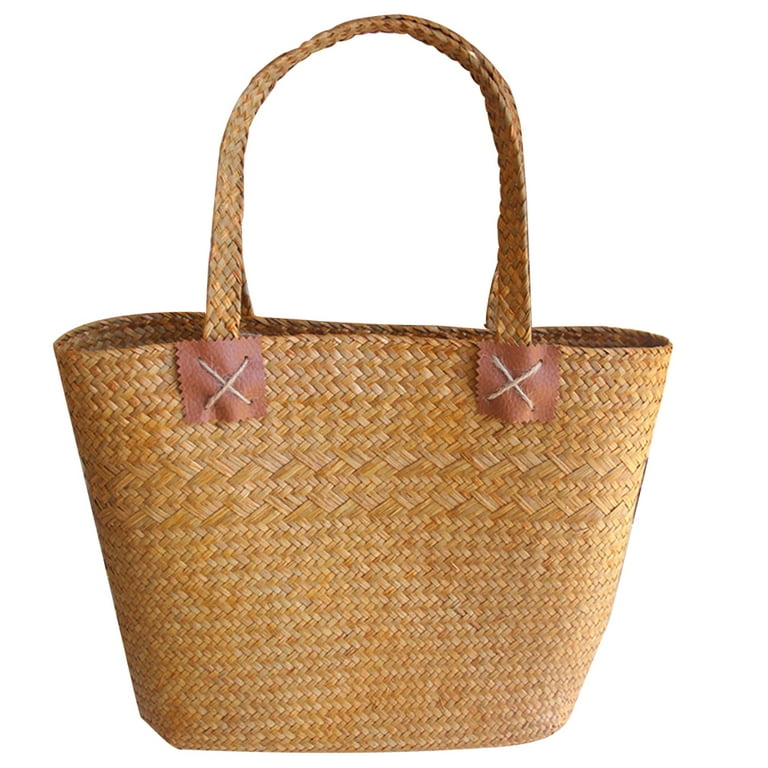The image features a light tan wicker tote bag with no background, filling the entire photo, akin to an item you'd see while shopping online. The straw-material tote, with a light brown color reminiscent of wheat, has an oval, somewhat squishable shape. The bag is equipped with two straps designed to go over the shoulder, attached via small, square patches made of deeper brown leather. These patches are secured with prominent X-shaped cross-stitching, possibly in matching brown thread. A distinctive design element appears about a third of the way down the bag, where the weaving transitions to a more intricate criss-cross pattern. This simple, yet functional and stylish beach or vacation tote exhibits a two-tone weave upon closer inspection, adding to its visual appeal.